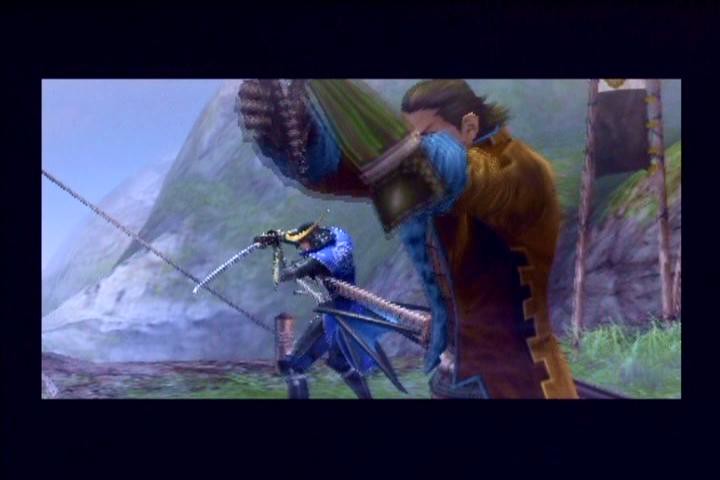In this captivating illustration set against a stark black backdrop, we are transported to the bygone era of pirates. The scene depicts two male figures, dressed in classic pirate attire, standing on a grassy hill. The man in the foreground commands attention with his ruffled blue shirt and brown jacket. His long brown hair flows freely, and although his face remains partially obscured by his arm, it is evident he is wielding a sword. His posture suggests he is poised for action, his arms raised as if in mid-motion.

Close by, another pirate figure enhances the scene with his distinctive attire. He dons a black and gold pirate cap, a blue jacket, and dark pants. His stance is assertive, holding a long silver sword pointed towards the west. The sword glimmers, hinting at its importance in the unfolding drama.

The setting adds depth to the illustration's historical richness. Water, tinted in dark gray, occupies the lower left corner, hinting at the proximity of the sea—an essential element in any pirate tale. Far off in the distance to the right, gray and green mountains rise, their rocky bases transitioning into verdant peaks, suggesting a rugged yet lush terrain. This detailed composition marries action and environment, enveloping the viewer in a vivid reenactment of a pirate's world.